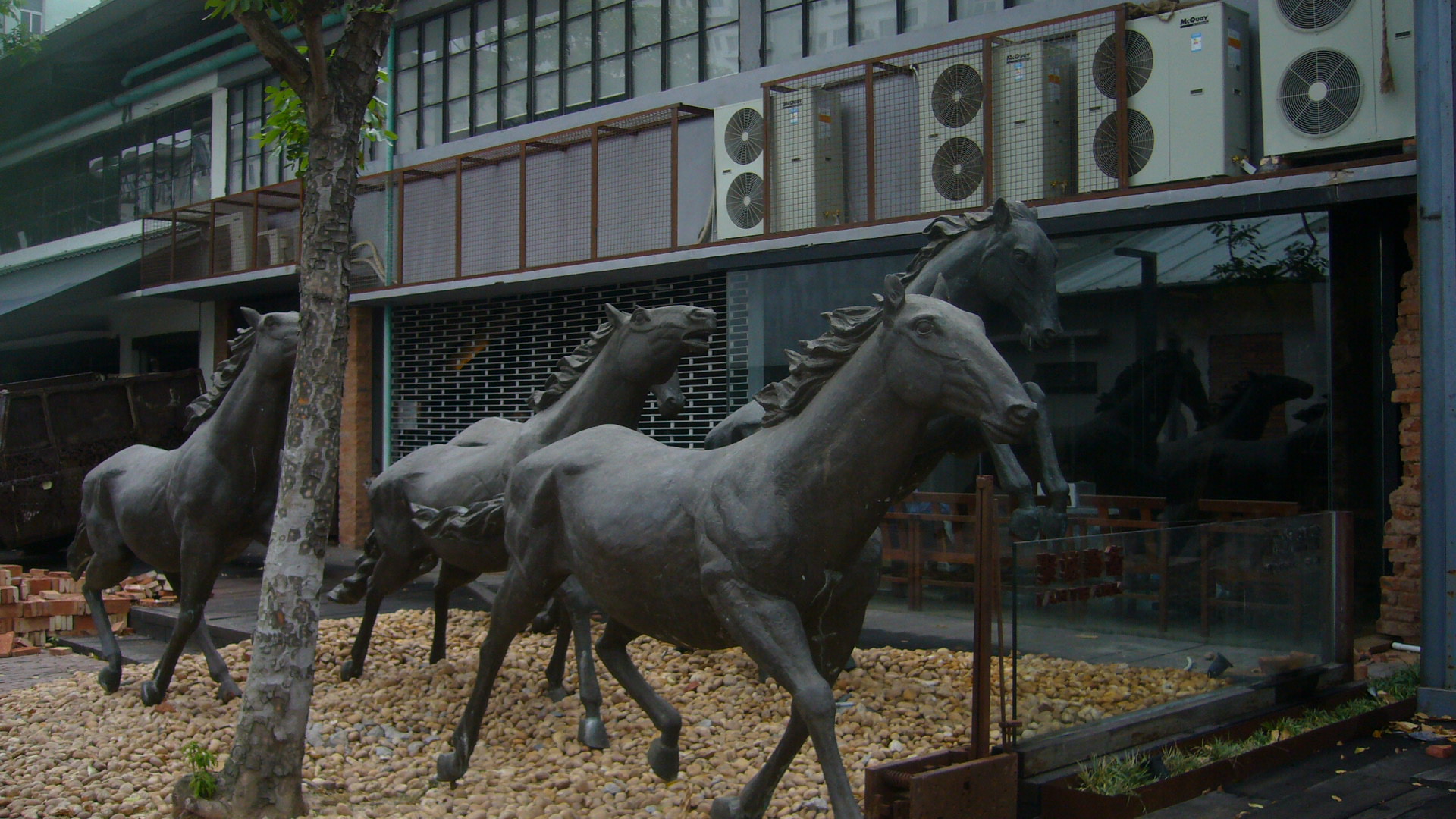This image showcases an outdoor art installation featuring life-sized statues of four wild horses in motion. Crafted from a dark, weathered bronze metal that appears almost blackish-gray, these sculptures vividly capture the horses' dynamic energy. Positioned in a courtyard covered with light-colored tan pebbles or stones, the leading horse is depicted with its mane and tail streaming as if blown by the wind, exuding a sense of momentum and freedom. Each horse is aligned from left to right, with the second horse seemingly leaping mid-air, front hooves raised, as if about to hurdle a low glass fence edged in iron. The third horse's expression appears slightly frightened, while the fourth is partly obscured by a gray tree trunk, making its features harder to discern.

In the backdrop, there are two storefronts—the nearer one partially visible behind a plate glass window and metallic security gate, possibly an idle restaurant with air conditioning units on its roof. The other storefront is further back, closed off by a metal grate. Additional details, like the sidewalk paths and areas of broken bricks near the stores, complement the scene, enhancing the realism and setting of this striking sculpture ensemble.